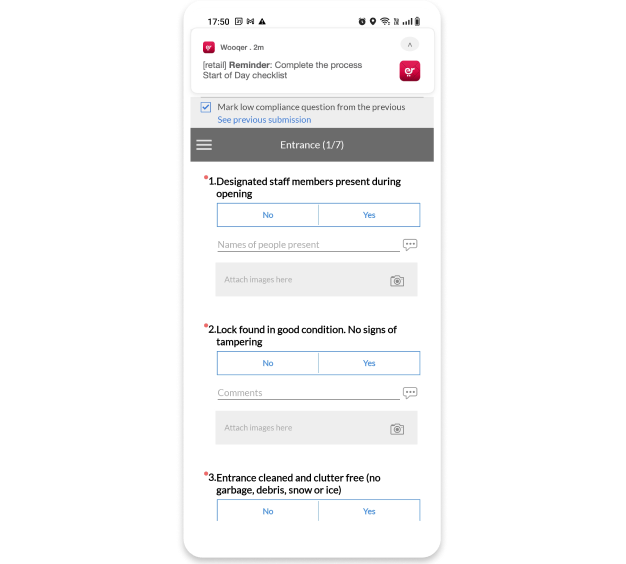Screenshot of Employee Checklist on Wooqer App

This detailed screenshot captures an employee checklist from the Wooqer app (spelled W-O-O-Q-E-R), displayed on an Android phone. At the top of the screen, the Android status bar shows the date, time, and various notification icons including an alarm, location services, Wi-Fi and data signals, and battery level, all in black.

Just below the status bar, there's a notification featuring the Wooqer logo, which is a red square with a white snail-like animal in the center. The notification is labeled "[Retail] Reminder" in bold letters, prompting the user to "Complete the process of Start of Day Checklist."

The app interface displays a gray rectangle with black text stating "Mark low compliance question from the previous session," alongside a blue checkbox and the option to "See previous submission" in blue text.

Beneath this, there is a darker gray rectangle with a three-bar menu icon on the left and white text stating "Entrance 1/7." This section is part of a menu in the app.

The checklist itself comprises several items, each marked with a red asterisk next to a numbered bullet point:
1. "Designated staff members present during opening" in black lowercase text. Options to select "No" or "Yes" are provided in blue-outlined rectangles, with blue text. Below this item is a blank gray line labeled "Names of people present," intended for the user to enter colleagues' names, accompanied by a speech bubble icon. A light gray rectangle beneath it displays "Attach images here" with a camera icon.
2. "Lock found in good condition. No signs of tampering." This item also has "No" and "Yes" options in blue-outlined rectangles with blue text. A gray line labeled "Comments," and a speech bubble icon are below this, followed by another light gray rectangle stating "Attach images here" with a camera icon.
3. The third bullet point, partially cut off, reads "Entrance clean and clutter-free. No garbage, debris, snow or ice." Below this text is a partial view of the same "No" or "Yes" rectangle.

The comprehensive details in this employee checklist are designed to ensure thorough and precise daily operations within the app.